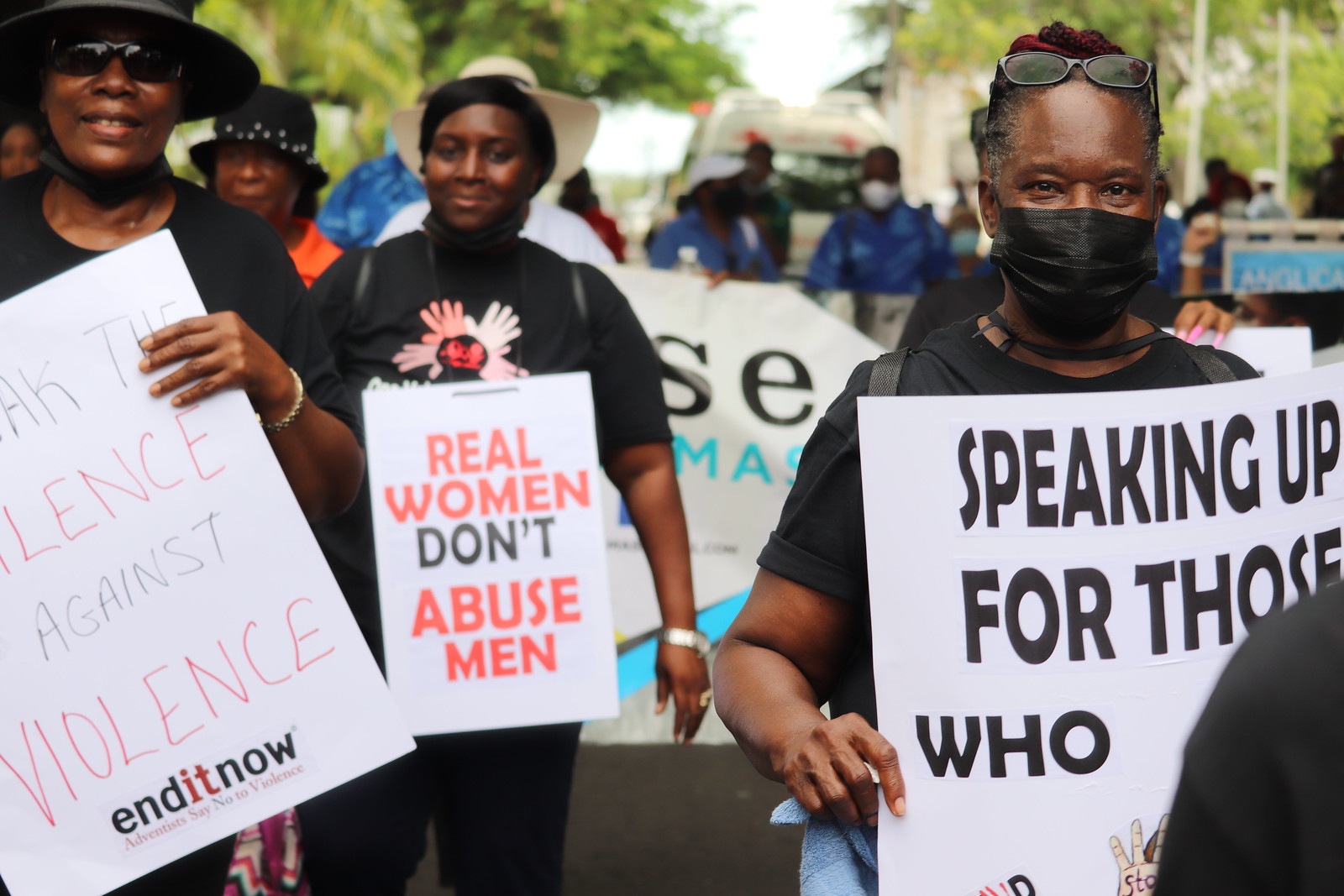The image depicts a diverse group of African American women participating in a protest rally or parade against violence. They are walking down a road holding various signs with different messages. In the forefront, there is an older woman wearing a black mask and glasses over her forehead, holding a white sign with black text that reads, "Speaking up for those who," though part of the sign is obscured by another person’s shoulder. To her right is a younger girl in a black shirt and black pants with a flower design, wearing a black cap and holding a sign that states in pink letters, "Real women don't abuse men." Another woman in the foreground, also wearing a black t-shirt and sunglasses, carries a sign with partial text visible, including, "violence against violence, end it now." The background features other protestors, but they appear blurry and indistinct. It is a daytime scene with trees visible in the background. An ambulance can also be seen further down the road behind the group.